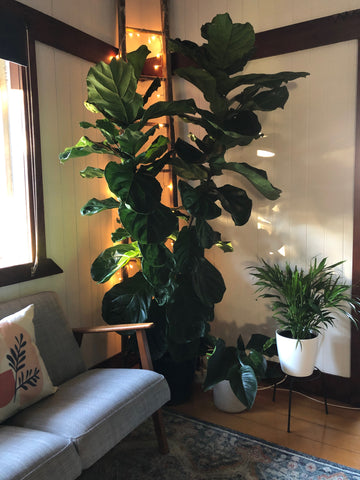This image captures the cozy corner of a room, drawing immediate attention to a towering houseplant that stretches nearly to the ceiling, showcasing its abundant, large green leaves. The Scandinavian-style loveseat with a grey cushion and a charming white decorative pillow resides to the left, partially visible and framed in an elegant wooden structure. The room itself is adorned with white paneling on the walls, accented by brown molding and floorboards, imparting a warm, minimalist aesthetic. Subtly illuminating the space is an orange runner light positioned behind the tall plant, creating a soft glow. Additional greenery adds to the atmosphere; a small fern perches on a black table to the right, beside another robust leafy plant nestled in a white pot. A window behind the sofa allows natural light to stream in, completing the serene and inviting scene.